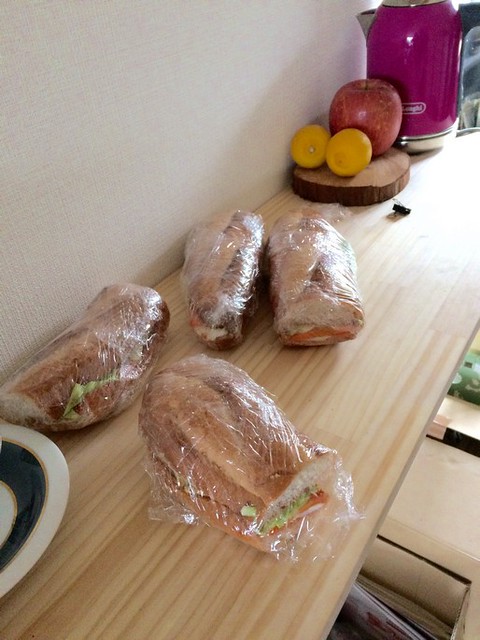The photograph captures a tidy display of four prepared and wrapped sandwiches lying on a wood grain synthetic surface, likely in a sandwich shop. Each sandwich, encased in clear plastic wrap, reveals layers featuring a high-quality, thick, and irregular bun, with visible tomato slices, lettuce, onions, ham, and possible traces of mayonnaise. The sandwiches are arranged diagonally and back-to-back on a shelf that runs from the bottom left to the mid-upper right of the image, against an off-white wall. Behind the sandwiches, at the far right end of the shelf, stands a magenta-colored electric teapot next to a wooden coaster holding a large red apple and two small lemons. Additionally, a partial view of a plate is visible at the bottom left, and there is a hint of a black object and some drawer space with books also present in the scene. The setting is cozy and orderly, indicative of a well-kept sandwich shop.